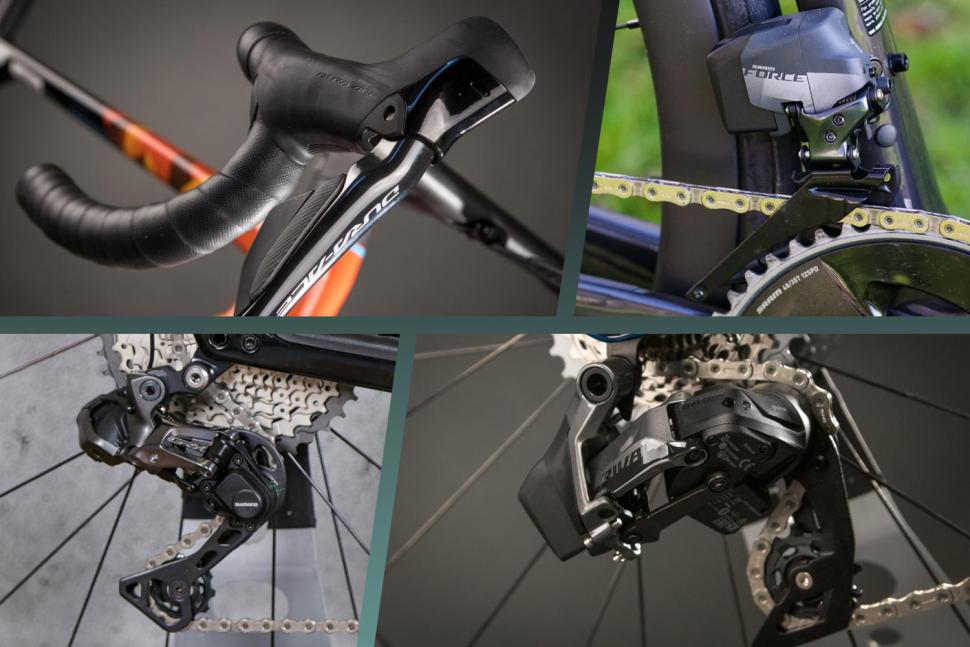This image is a composite of four photographs showcasing various components of a road bike against a gray and white backdrop. 

- The top left photo features a black handlebar with an attached brake lever, displaying the text "Dura-Ace" in white vertically. The handlebar faces the bottom right, and in the softly blurred background, parts of the bike frame can be seen in black and orange.
  
- The top right photo highlights the front derailleur, labeled "SRAM Force." The derailleur is a mix of taut gray and light gray with a black body, accompanied by a bike chain running through it. A wheel is also visible behind this component.

- The bottom left image depicts the rear derailleur, which is black and ensconced in a silver, S-shaped device that holds the bike chain. Silver spokes of the bicycle wheel are visible in the background.
  
- The bottom right photo provides another perspective of the rear derailleur, focusing on a clean, metallic small engine with black gears, shot from the bottom up. This component also features visible bike spokes in the background.

Each image is bordered by a dark blue frame, enhancing the contrasts and details of the bicycle parts within.